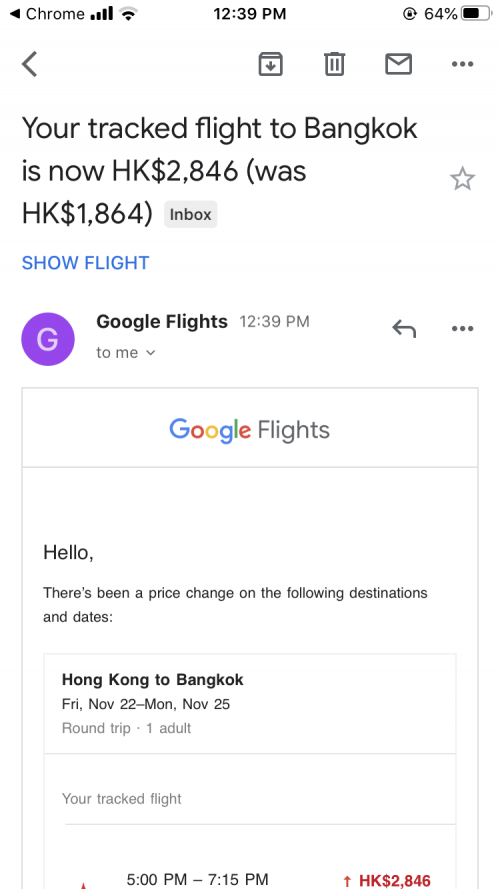The image is a detailed screenshot captured from a mobile device, which displays an email notification within the Chrome browser. The screenshot shows a full carrier signal with four bars and a moderately weak Wi-Fi connection with two bars. The time on the device is 12:39 p.m., and the battery level is at 64%.

In the email content, various navigation icons are seen at the top, including a back button, a save button, and a trash button. The primary message of the email, written in black text, indicates a flight update: "Your tracked flight to Bangkok is now HK 2846, was HK 1864." A gray star button is also visible, which might be a bookmarking feature. Additionally, a blue hyperlink labeled "Show flight" invites the user to view more details.

Embedded within the email, there is a recognizable purple Google logo, signifying the email is from Google Flights. Below the logo, in black writing, it reads "Google Flights." The body of the message states: "Hello. There's been a price change on the following destinations and dates: Hong Kong to Bangkok, Friday, November 22nd, through Monday, November 25th, round trip for one adult, leaving at 5 p.m. to 7:15 p.m."